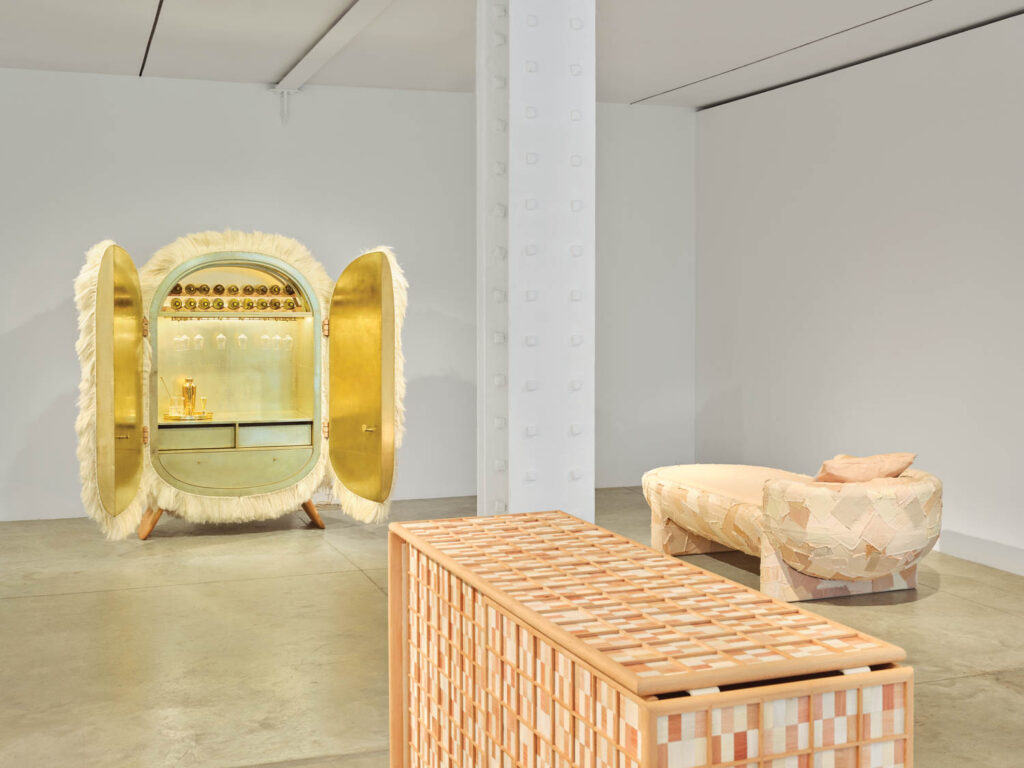This color photograph captures the interior of a room that closely resembles an art gallery. Dominating the scene is a prominent white, square pillar positioned centrally against a backdrop of pristine white walls and ceiling, which create a stark, clean aesthetic. The floor is polished concrete in beige and gray hues, adding an industrial touch to the setting.

On the left side of the image, there's an elaborate armoire with two open doors, covered in pale yellow faux fur. The interior of this armoire gleams with a metallic gold finish and doubles as a sophisticated bar setup. Inside, there are gold bottles displayed horizontally, wine glasses hanging elegantly from a shelf, and a gold drink shaker accompanied by various bar accessories on a lower shelf.

To the bottom left of the image, there's a golden and white cabinet with a fashionable design, resembling a dresser with multiple drawers. At the center of the room, a prominent decorative piece captures attention: a large rectangular box adorned with a checkerboard pattern in peach and white tones, perhaps suggestive of a paper-mache texture.

On the far right, a luxurious chaise lounge stretches out, crafted from materials that give off a peachy hue with subtle gray and light pink squares woven in. Topping off this stylish piece is a matching pink pillow, enhancing the cohesive and sophisticated color palette of the room.